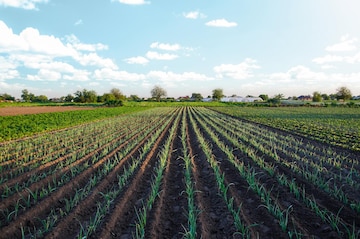The image is a detailed color photograph of a farm taken from a slightly elevated perspective. The main focus is on a series of tilled and planted fields, with neatly organized, alternating rows of crops and dirt paths. The crops are young, short, and green, resembling plants like onions or corn, but the type remains unclear. These plants are sprouting from small mounds and are growing close together. Surrounding the central rows of crops, on either side, are fields of green grass and patches of dirt. Towards the left, there lies a muddy area, hinting at recent plowing or rainfall. In the distant background, a line of trees and a few indistinguishable buildings, possibly greenhouses, can be seen. The sky above is a pale blue, fading lighter towards the horizon, with scattered fluffy white clouds, creating a serene rural landscape.